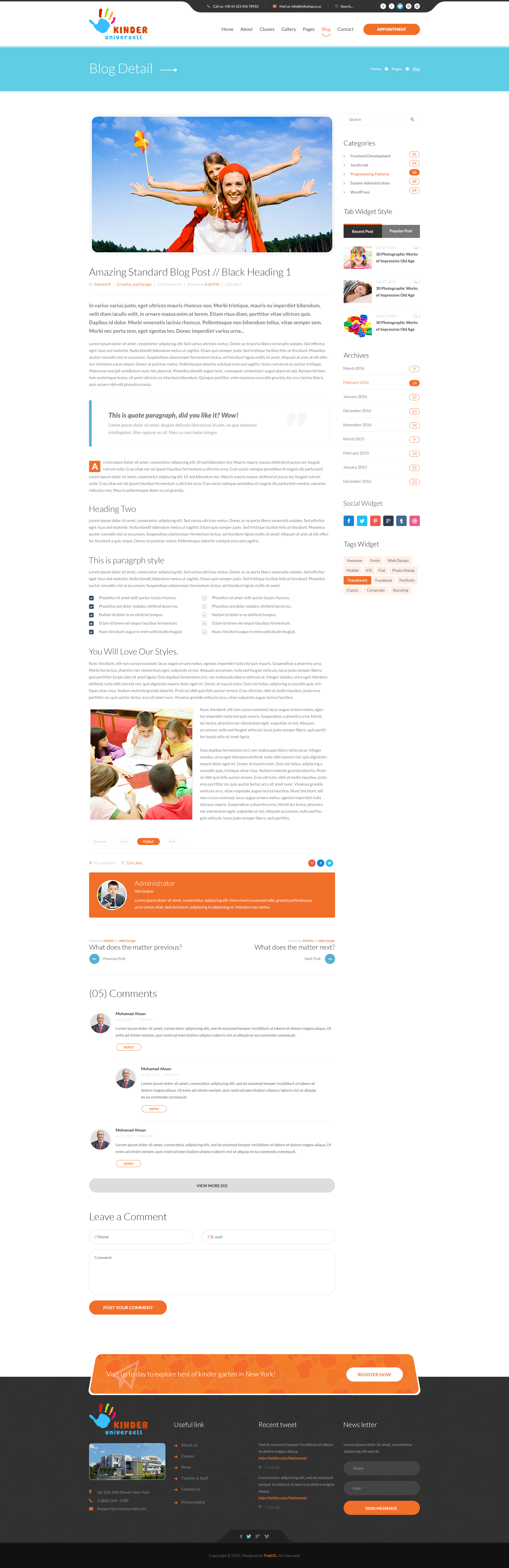This image is a screenshot from a mobile device displaying a website that appears not to be optimized for mobile viewing, with very small and difficult-to-read text due to the zoomed-out perspective. The overall color scheme of the site includes blue, orange, and white, with the background space primarily white. Dominating the top left corner is a logo featuring a multi-colored handprint. The palm and thumb are blue, while the fingers range from orange, yellow, to green hues. The logo text reads "Kinder Universal," stylized as "Kinder Universell."

At the top of the webpage, there is a navigation bar with tabs labeled Home, About, Classes, Gallery, Pages, Blog, and Contact. An orange button labeled "Appointment" is prominently positioned nearby. Just below this, a blue banner reads "Blog Detail," accompanied by a decorative right-pointing arrow.

The main body of the page features an image of a woman carrying a young girl on her back, both mimicking airplanes with their arms spread wide. The girl holds a small paper fan toy in her right hand. Below this image, there is an extensive amount of text, likely making up the blog content, followed by another image and several comments. On the right side of the page, there are recommendations and links to other sections of the website.